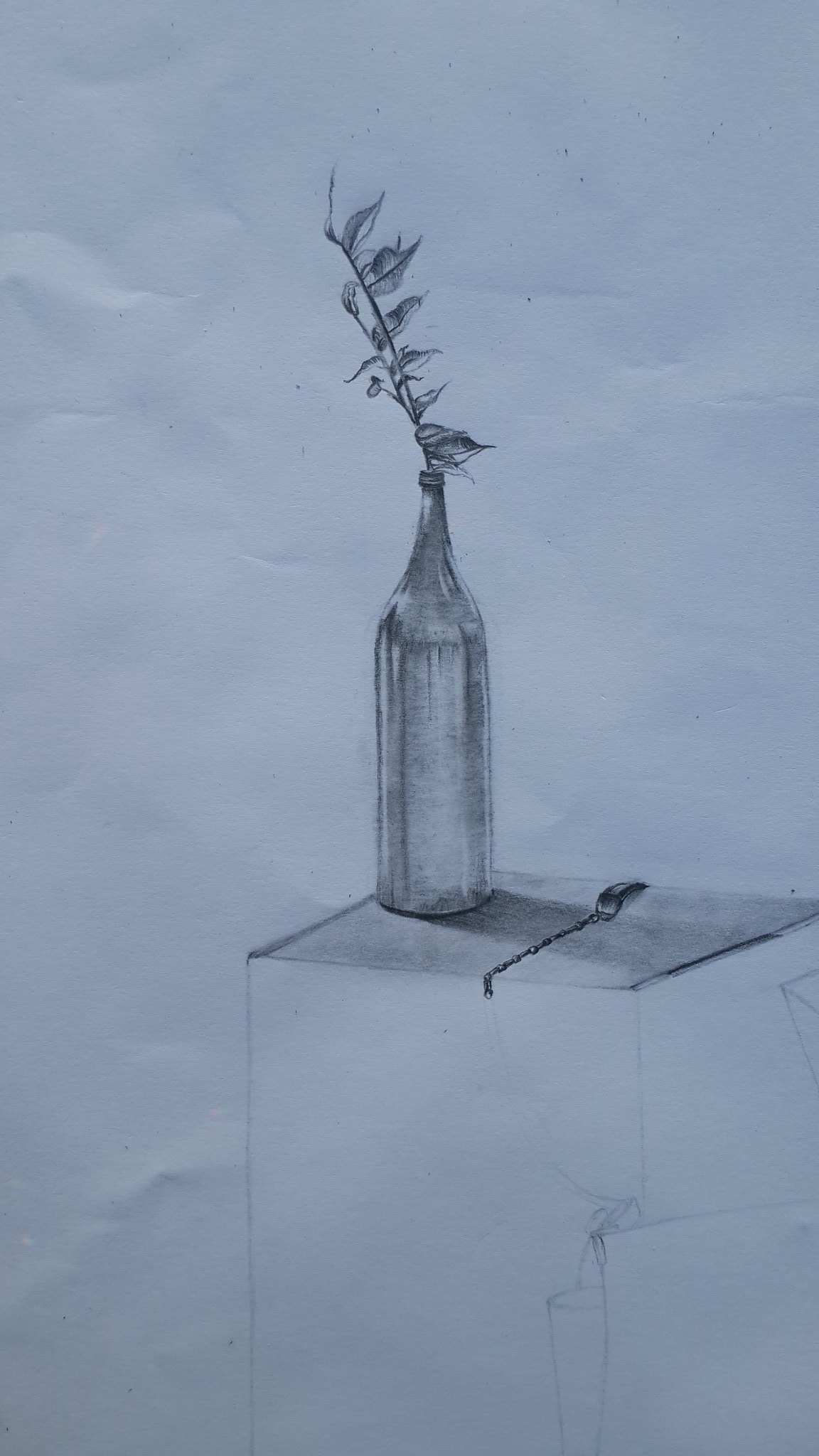A detailed pencil sketch on a wrinkled white paper depicts a bottle resting on a countertop. The bottle is intricately shaded, giving it a realistic three-dimensional appearance. To the right of the bottle, there’s a section that resembles a bucket. An ornate chain drapes across the scene, adding a touch of texture and complexity. From the top of the bottle, a flower sprouts elegantly, with darkly shaded branches and leaves extending outward. The leaves are particularly prominent, extending to the upper right, accentuating the intricate details of the drawing.